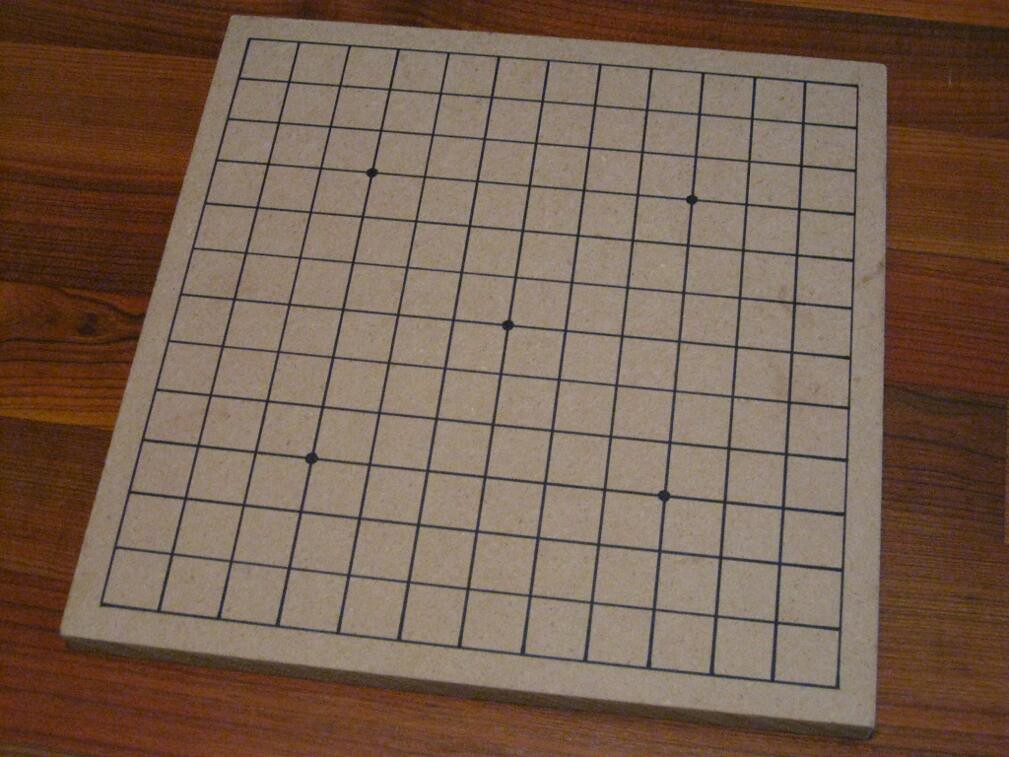The image depicts a square game board, likely made of beige wood or a plywood-like material, featuring a meticulously drawn grid of 12 by 12 black squares, totaling 144 squares. Prominently, five dots are placed within the grid: one centrally located and four others equidistant from the center dot towards each diagonal, resembling the arrangement on a number five face of a die. The board is slightly tilted to the right and rests on a dark brown surface, which appears to be either a wooden floor or possibly luxury vinyl, though its exact size cannot be determined from the image alone.